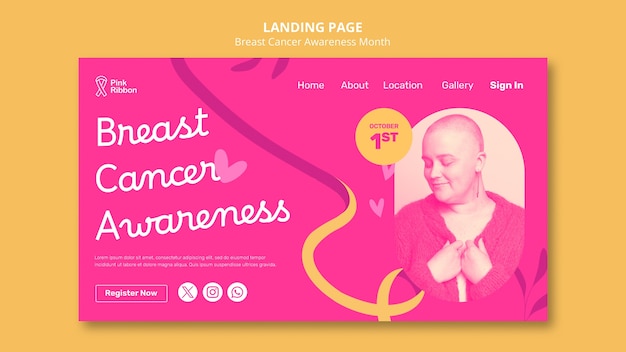The image displayed on the website features a vibrant, orange background with a central rectangular section in pink that dominates the landing page, promoting Breast Cancer Awareness Month. Positioned slightly to the left within the pink rectangle, the phrase "Breast Cancer Awareness" is elegantly written in white cursive lettering, accompanied by a small pink heart next to the word "cancer." The visual centerpiece is a touching photograph of a woman, who appears to be smiling softly with her eyes closed. She is seen with her hands near her heart, wearing a V-neck sweatshirt, and exhibiting a gentle, serene expression. Her head is slightly turned to the left, revealing a close-cropped hairstyle that almost appears as a light fuzz. Above the image, navigation options are clearly visible, including links labeled "Home," "About," "Location," "Gallery," "Sign In," and the date "October 1st." The overall design emphasizes empathy and support, reinforcing the theme of breast cancer awareness.